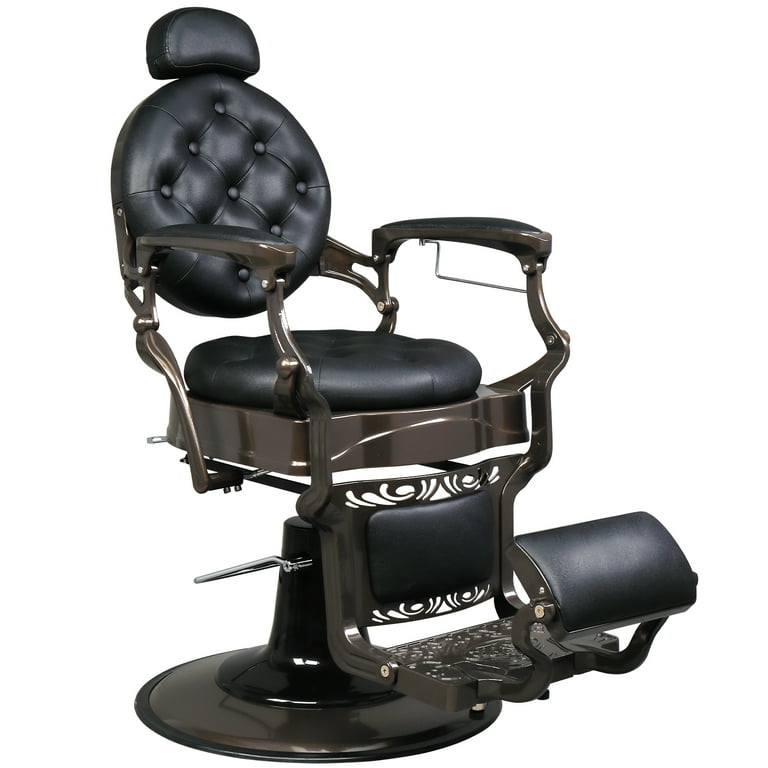This photograph features an antique chair, possibly from an old barber shop, dentist office, or shoeshine stand, set against a white background. The chair sits on a black pedestal base and features a robust round seat and back, both upholstered in black leather or leather-like vinyl. The back of the chair includes a small, half-moon style headrest. The chair also has stainless steel armrests that are partially covered in matching black leather upholstery.

A key characteristic is the chair's ornate metalwork, especially around the footrest and the base's scrolling designs. A thick metal footrest with intricate designs extends from the lower part of the chair, providing an area for foot support, including an additional black leather section for higher foot placement. The lever on the back allows the chair to be tipped backward, enhancing its functional design. Overall, the chair combines aesthetic elegance with practical features typical of vintage service furniture.